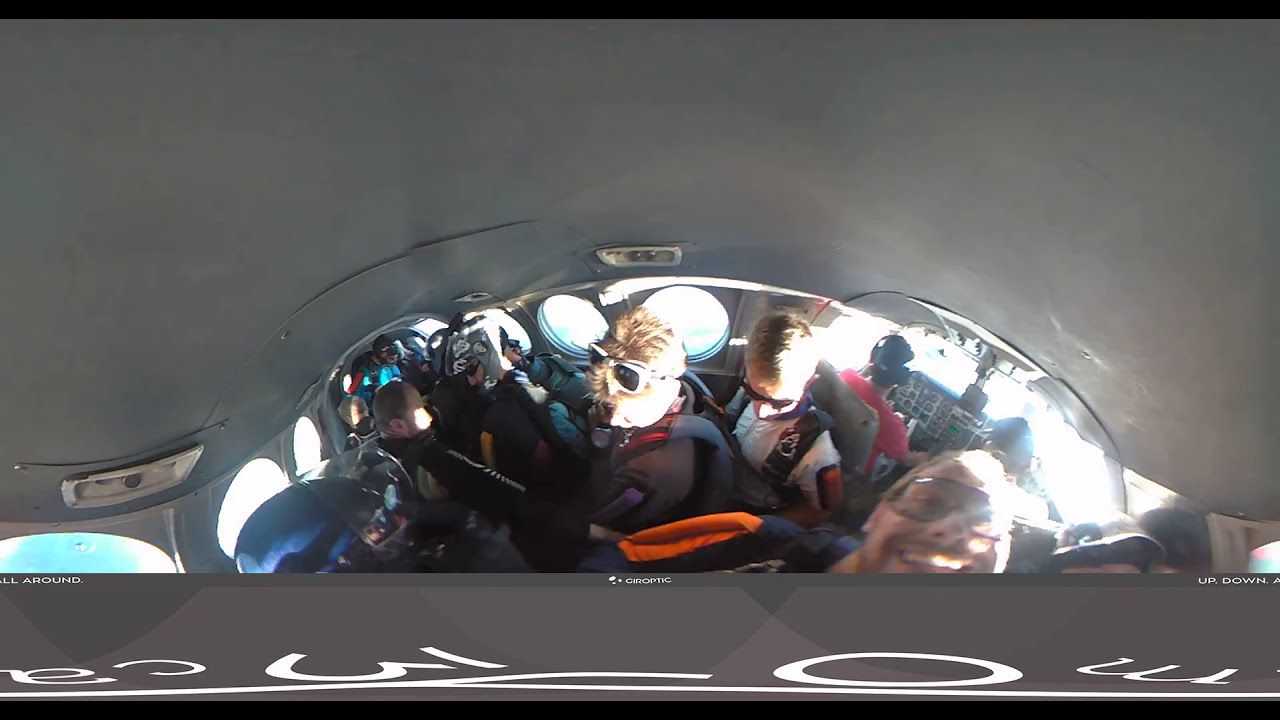This horizontally aligned panoramic image, framed with a thin black border at the top and bottom, captures the lively interior of an aircraft preparing for a skydiving adventure. The smooth gray ceiling of the small airplane cabin is visible as the wide-angle lens encompasses nearly the entire group of about 10 to 15 skydivers. Most are gearing up with parachutes strapped to their backs, clad in skydiving uniforms, helmets, and some with goggles. In the cockpit, located on the right side of the image, the pilot with a red shirt, headset, and a black ball cap can be seen, likely steering the plane accompanied by a possible copilot. A standout figure in the lower right corner, wearing goggles and smiling broadly, appears to be taking the photo, creating a dynamic and engaging perspective where some people in the group are looking towards the camera. The arrangement offers a clear view of both the cockpit at the front and the tail of the plane at the back, effectively capturing the anticipation and excitement of the skydivers ready for their jump.